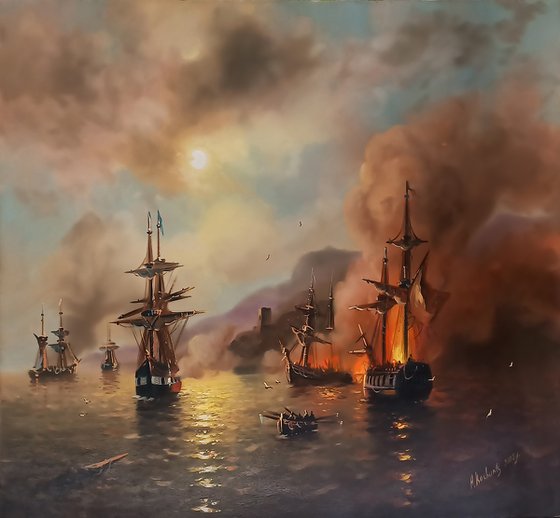The image is an oil painting depicting a dramatic maritime scene. In a dark, stormy-looking sky that is starting to clear up, clouds of dense smoke rise from at least two ships on fire situated toward the right of the composition. Bright orange flames can be seen shooting off the burning vessels, casting a noticeable yellow and orange glow into the sky and reflecting dramatically on the dark gray ocean water below. Amidst the chaos, smaller rowboats can be seen on the water, including one in the foreground with oars raised high and at least five figures aboard, possibly escaping from the fires. The calmer waters, despite some white caps and waves, add contrast to the turbulent atmosphere created by the burning ships. Additional ships with upright masts, unaffected by the fire, are scattered towards the left, while the light blue sky and yellow sun in the background hint at the storm's passing. A partially legible signature of the artist appears in light gray at the bottom right of the painting.